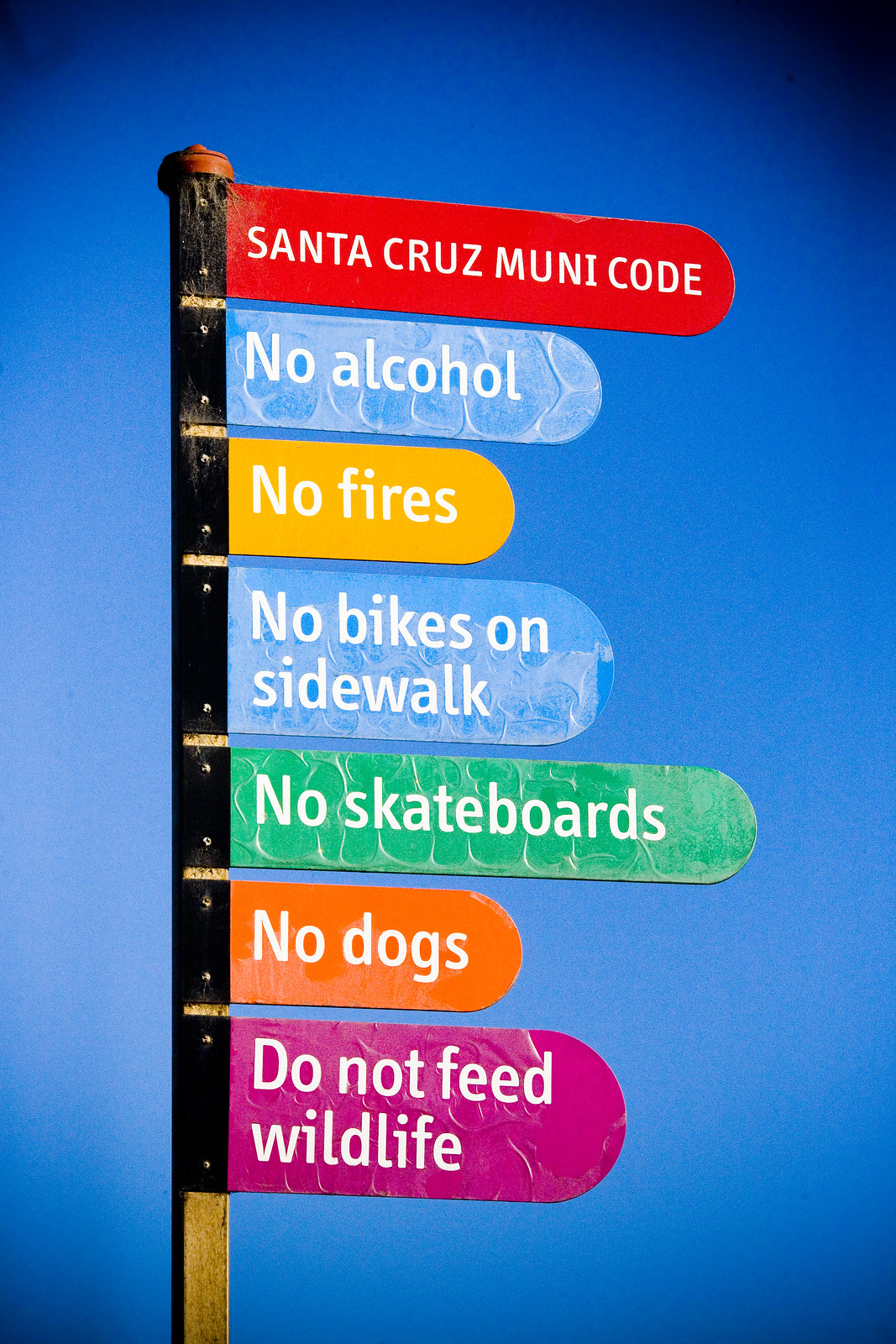The image displays a tall, slender wooden signpost, topped with a small nub or knob. This signpost stands against a vivid blue sky backdrop, with a noticeable vignette effect that darkens the edges at the top and lightens them at the bottom. Affixed to the right side of the post are seven small, rounded rectangular panels, each with distinct background colors and clear white sans serif text, listing various municipal regulations. The topmost panel is red and reads "Santa Cruz Muni Code" in capital letters. Beneath it, the second panel is blue and states "No Alcohol." The third panel is yellow and says "No Fires." The fourth panel, also blue, announces "No Bikes on Sidewalk." The fifth panel is green and declares "No Skateboards." The sixth panel is orange and prohibits "No Dogs." The bottom-most, seventh panel is pinkish-purple and commands "Do Not Feed Wildlife." Each panel is securely attached to the pole with black screws at the top and bottom.